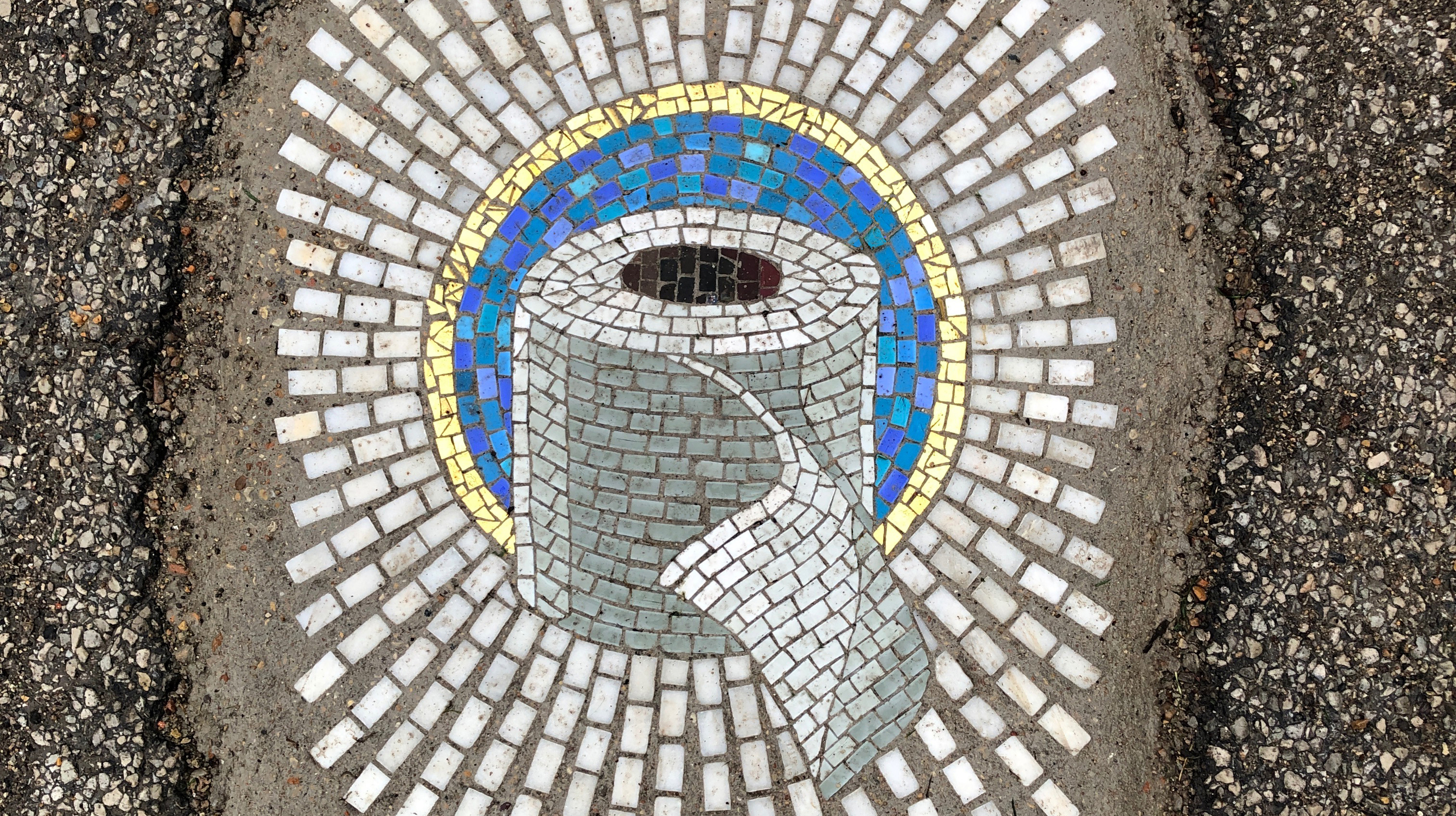In this outdoor photo, the focus is on an intricately crafted mosaic set into a pothole in a gravelly road. The mosaic reveals an artistic depiction that echoes the design of stained glass one might see in a cathedral. Dominating the center of the mosaic is a prominent roll of toilet paper, standing upright with the black interior core visible from above. Radiating outwards from the toilet paper is a striking blue disc, which is bordered by a golden ring. This blue-and-gold centerpiece emits white lines in a mosaic pattern, creating a burst effect that extends towards the edges, blending into the surrounding gravel and mud. The dull asphalt and dirt surrounding the mosaic indicate it has been cleared to showcase this unique piece of urban artwork, devoid of any people or text.